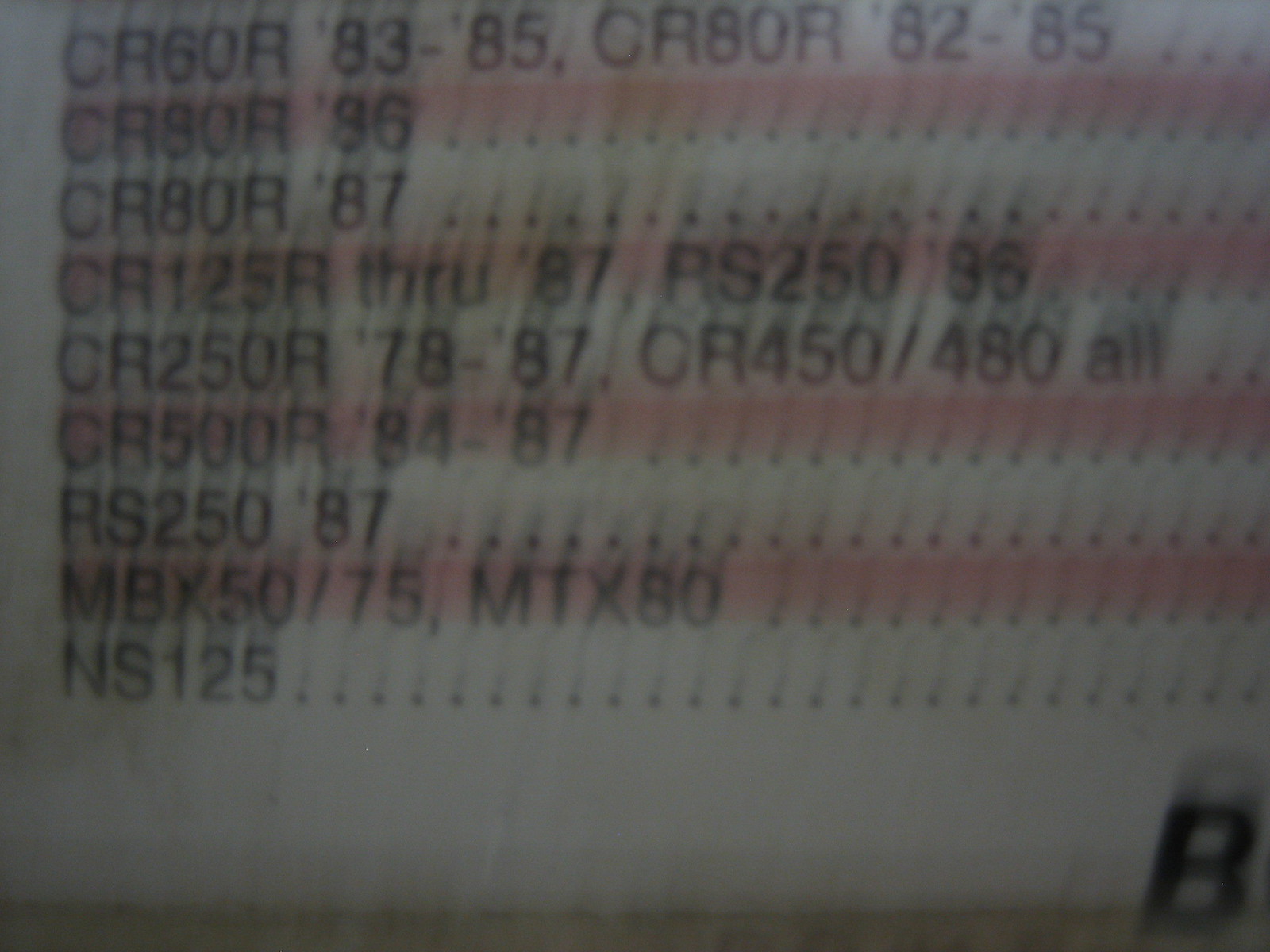Here is a cleaned-up and detailed caption based on the provided description:

---

This image features a slightly blurry, typed list of numbers and parts, displayed on a white piece of paper. The text is in black lettering, providing high contrast against the white background. Red lines outline and separate each row, enhancing readability. Each row concludes with a series of light gray dots. The text progresses from top to bottom as follows: 

1. CR060R 83 to 85, CR80R 82 to 85
2. CR80R 86, CR80R 87, CR125R through 87, RS250 86
3. CR250R 78 to 87, CR450/480 all
4. CR500R 84 to 87
5. RS250 87
6. MBX50/75, MTX80
7. NS125

On the far bottom right corner of the paper, there is a large black letter "B," which appears slightly blurred.

---

This revised caption provides a structured and detailed overview of the image content.